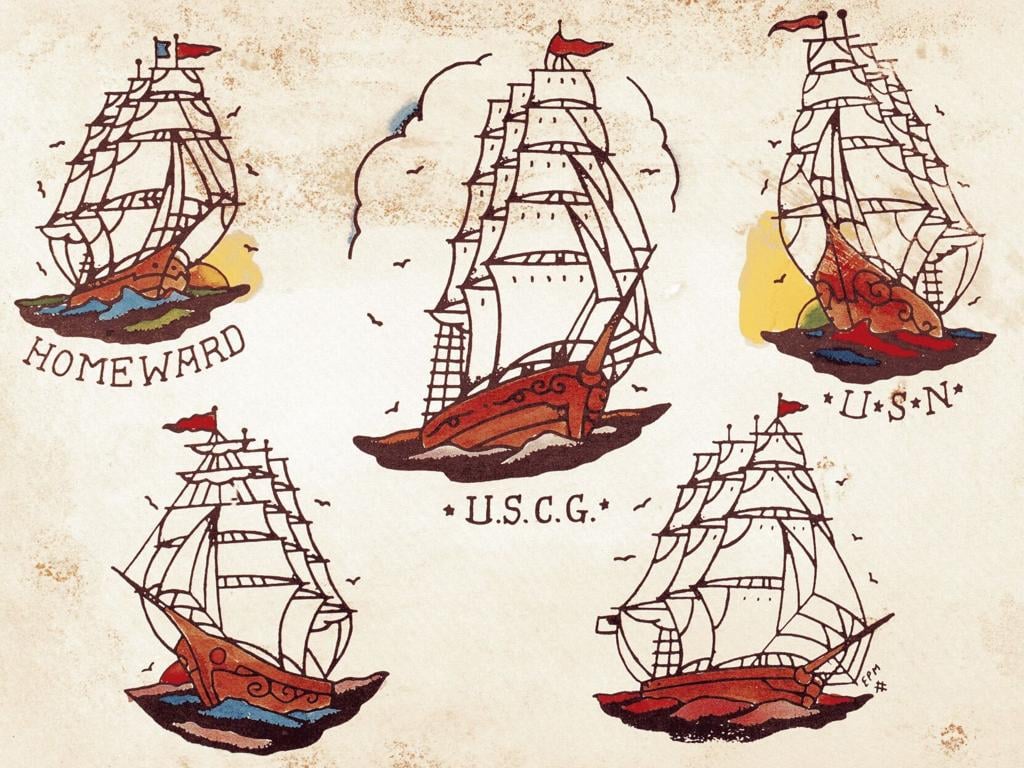This image showcases five detailed, old-fashioned illustrations of sail ships. The background, an aged, off-white paper with splotches of reddish-brown, enhances the vintage appearance of the artwork. Each ship is rendered in meticulous detail, with brown-toned line work that defines their wooden structures and numerous white sails. 

The top row features three ships: the leftmost ship is labeled "Homeward" and is adorned with a blue and red flag. Next, the largest ship at the top center is marked "USCG," suggesting it belongs to the U.S. Coast Guard, and has a single red flag. To its right, a smaller vessel labeled "USN" represents the United States Navy and also flies a red flag. 

Two more ships occupy the bottom row; these are unlabeled, possibly having their names cut off. All five ships display striking triangular red flags atop their masts. Directionally, the "Homeward," "USCG," and bottom right ship face to the right, while the "USN" and bottom left ship face to the left. Delicately sketched birds and subtle cloud shapes add to the dynamic atmosphere, with the sea visible at the base under each ship. These substantial ships, equipped with extensive sails, allude to vessels built for long voyages.